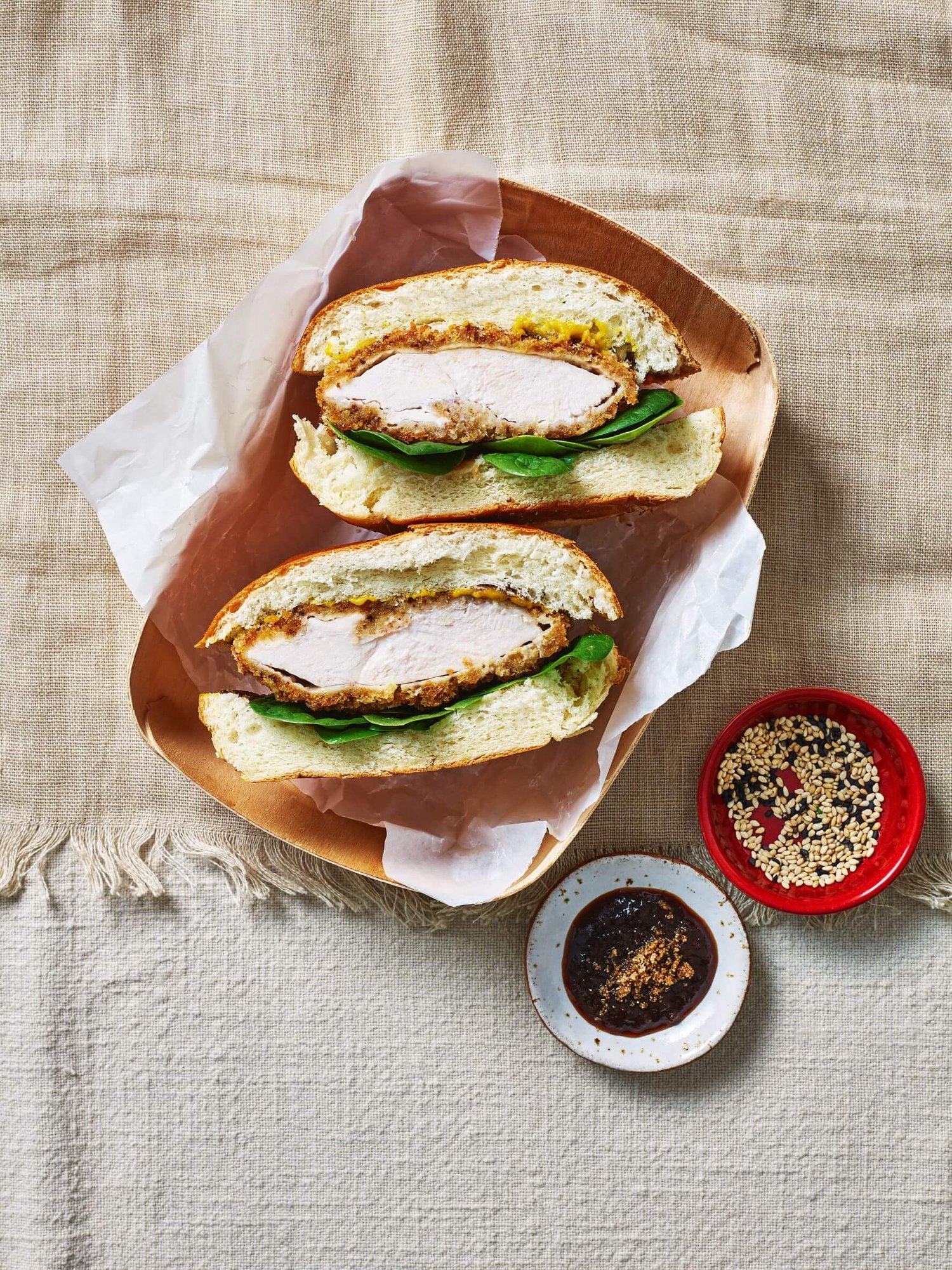This overhead photograph showcases a hearty sandwich nestled in a rectangular cardboard basket lined with parchment paper, adding a touch of fast-food nostalgia. The sandwich, cut in half with the cut sides facing upward, reveals the inner layers of a breaded and fried chicken patty. Below the sandwich, fresh spinach leaves provide a burst of vibrant green. The buns are golden brown on the outside with a soft white interior, topped with a dollop of yellow mustard spread across the chicken. To the right of the basket, two small containers sit on a rough white tablecloth. One container, red, holds a mix of black and white seeds, while the other, a white container, contains a brownish sauce with a sprinkling of tan seasoning on top. This meticulous arrangement highlights the fresh and inviting ingredients, making it a visually appealing and appetizing spread.